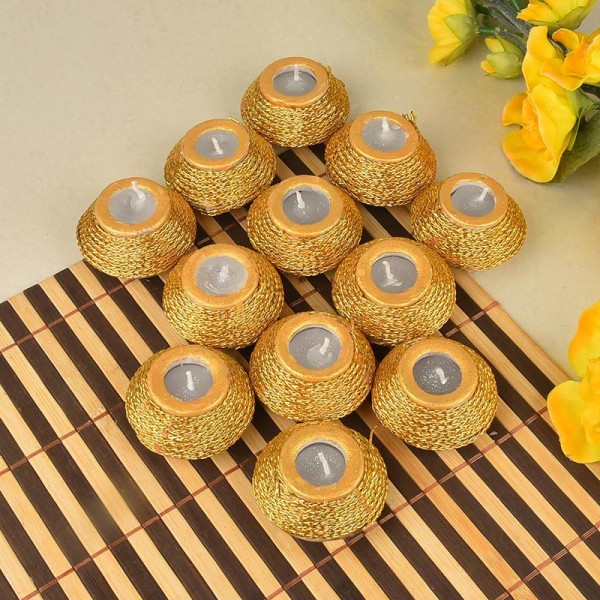In this image, an assortment of approximately a dozen circular candles is displayed prominently on a tan and yellow multi-colored mat, which is situated atop a cream or white-colored table, possibly in a kitchen or dining area. Each candle is held in a broad, golden brown holder that tapers at the top and bottom, giving them a burlap-like texture with a smooth top rim. The candles themselves are gray with white wicks, and they are all unlit. The arrangement of the candles forms a loose diamond shape: five candles on the top row, followed by rows of three, three, and one at the bottom. Additionally, in the top right corner of the image, there is a small bouquet of medium yellow flowers, with a few stray petals scattered in the bottom right. The mat under the candles is dark brown with light brown vertical stripes, possibly resembling wood slats bound with strings, further enhancing the rustic aesthetic of the scene. The overall color palette includes tan, yellow, green, gold, white, silver, black, and brown.